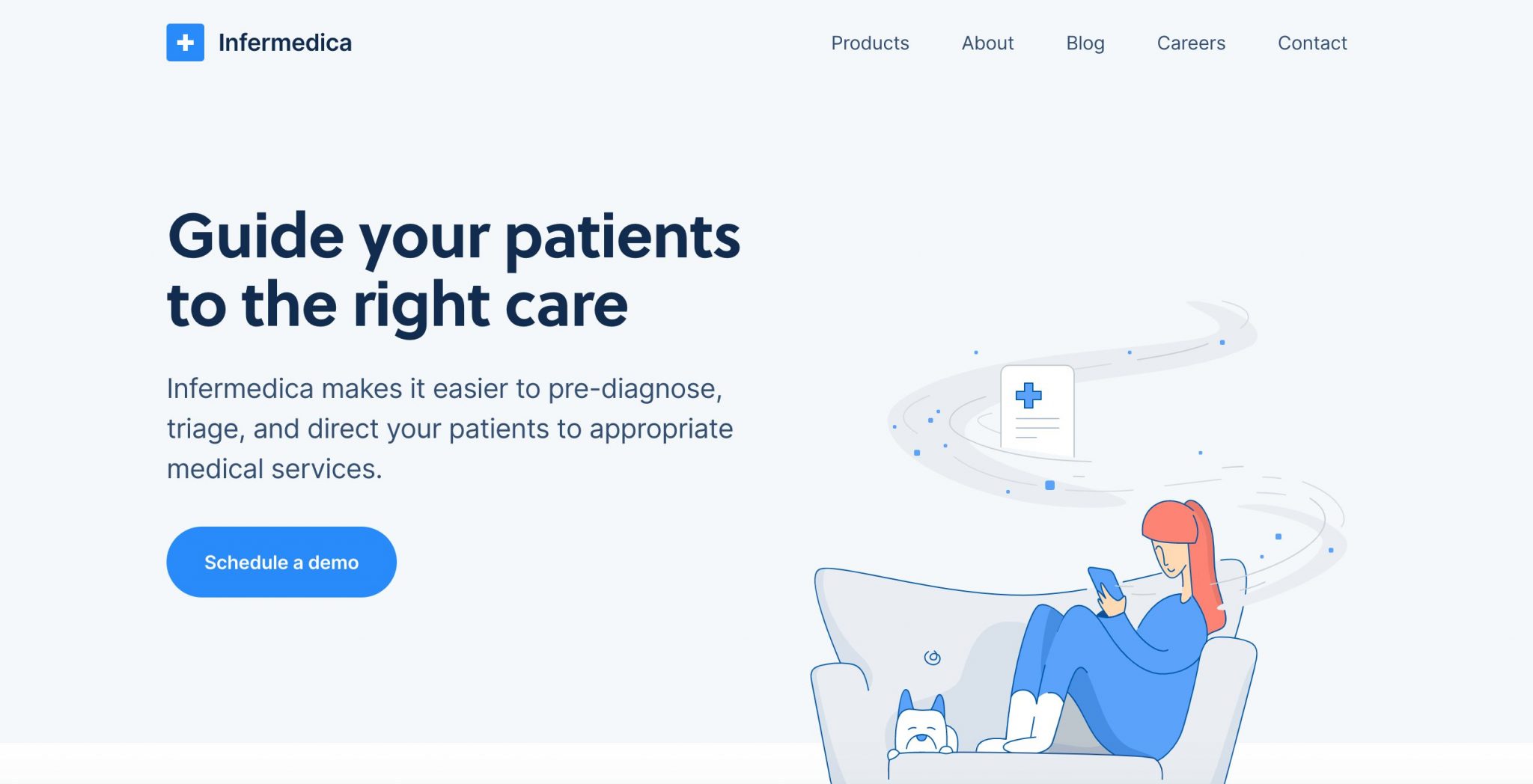This is a screenshot of the homepage of the Infermedica website, set against a light blue background that extends about an inch from the left. Prominently displayed on the left side is a blue circle containing a white plus sign. To the right of the circle, in bold black letters, is the brand name "INFERMEDICA."

At the top center, there is a navigation menu in smaller black lettering, listing links to various sections of the website: "Products," "About," "Blog," "Careers," and "Contact."

The bottom section features an illustration of a living room setup. On the left side of a light blue couch, a white dog with blue ears is sleeping, with its head facing the viewer. To the right of the dog is a woman facing left, looking down at her phone. She is dressed in an all-blue outfit with white socks and is sitting with her feet up on the seat. Her red hair flows dramatically upwards, creating a slightly chaotic look, accompanied by a hazy gray cloud. Encased within this cloud is a white square featuring a large blue plus sign.

Below this illustration, on the left side, bold letters proclaim, "Guide Your Patients." Adjacent to it, in smaller black text, a description reads: "Infermedica makes it easier to pre-diagnose, triage, and direct your patients to appropriate medical services."

At the very bottom, there is a conspicuous blue button with white text that reads, "Schedule a Demo."